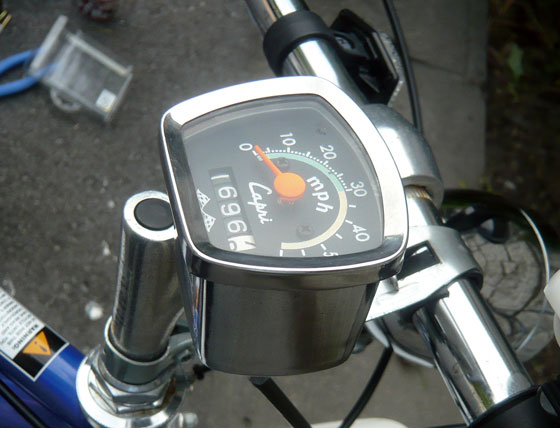A daytime outdoor photograph captures a close-up portion of what appears to be a bicycle. The focal point of the image is the chrome handlebars, adorned with a speedometer. The speedometer features a black face with white lettering and numbers, displaying speed in miles per hour and an odometer. Black wires snake around the handlebars, which also include attachments for headlights. A chrome bar extends downwards, connecting to a blue section of the bicycle frame. The ground beneath is concrete, bordered by a patch of dirt with a few scattered leaves. Additionally, some blue-handled tools, possibly pliers, lie blurred in the background.